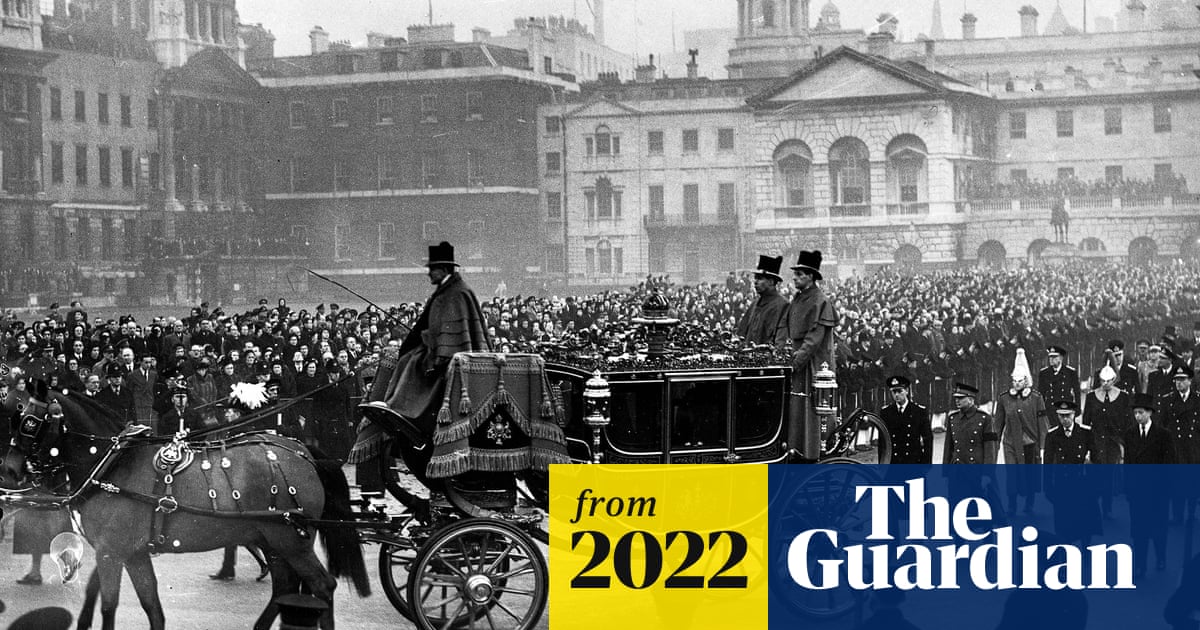This black-and-white image depicts a historical scene, likely from England or another European country. At the bottom right, text boxes indicate it was featured by "The Guardian" in 2022, with a yellow box displaying "From 2022" and an adjacent blue box saying "The Guardian." The central focus is an old-time hearse, a wagon drawn by two horses, with a driver at the helm. On the back of the hearse, two men are seen standing and holding on as it moves down a road. Behind the hearse, several uniformed officers parade, many of whom have distinctive military hats, including some with tall, pointed designs. The entire procession appears to be part of a funeral, as indicated by the somber atmosphere and the mass of onlookers lining the roadside, suggesting a significant public event. In the background, there are two contrasting buildings: a dark-colored brick structure and a lighter stone building, both framing the scene.